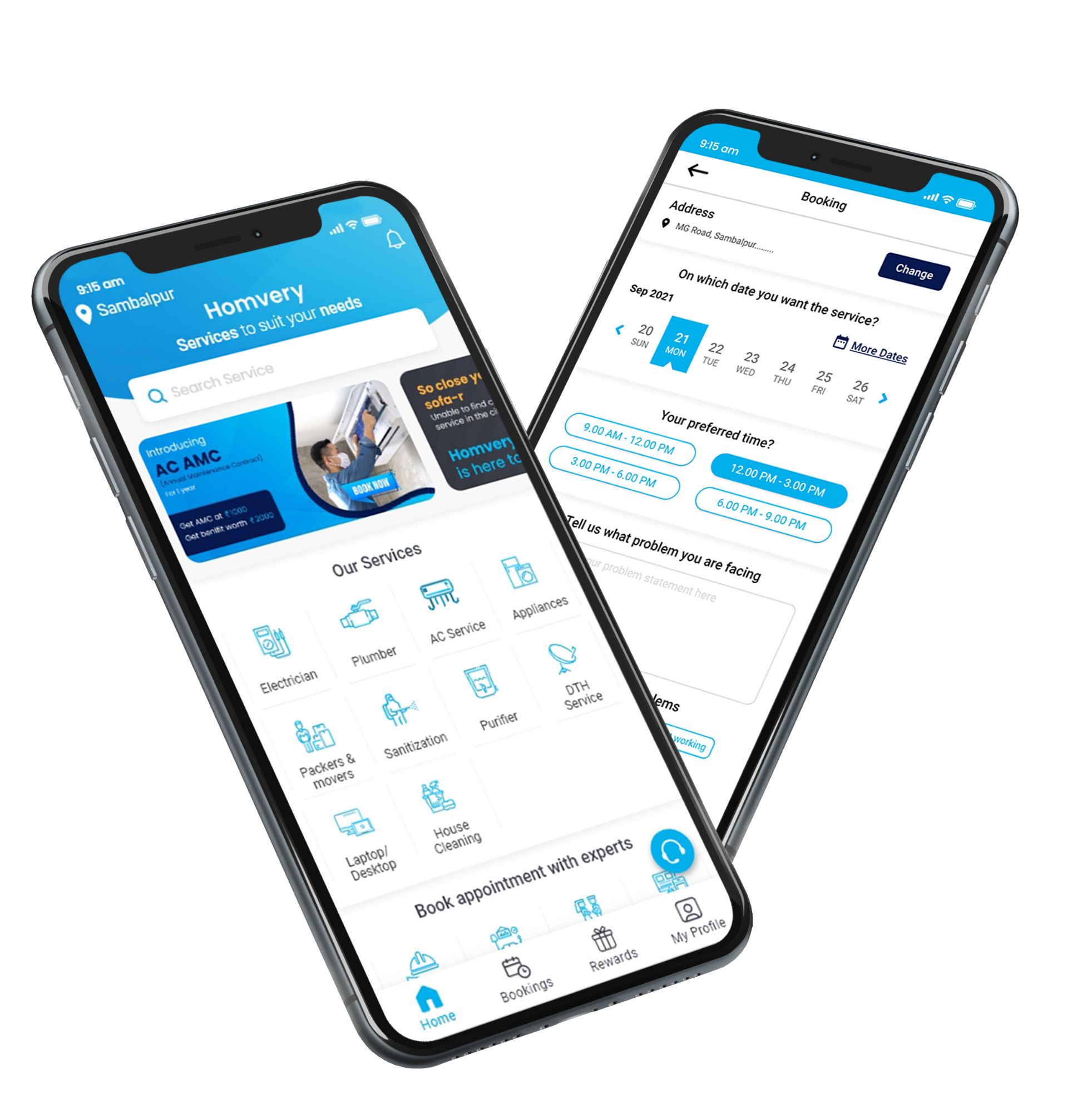The image features two smartphones positioned at varied angles, one slightly leaning in front of the other. The background of the image is predominantly white, creating a clean and uncluttered look that focuses attention on the phones themselves. Both screens display the interface of an app called Homevery, which is designed to offer a plethora of home and personal services.

The Homevery app, distinguished by its blue color scheme, showcases a list of available services such as electricians, plumbers, AC servicing, appliance repair, packing and moving assistance, sanitation services, water purifier maintenance, DTH service, laptop and desktop repairs, and house cleaning. The tagline "Services to suit your needs" is prominently displayed, indicating the app’s purpose of connecting users with various service providers.

The screen on the phone in the background shows a booking interface. It displays options for scheduling an appointment, specifically highlighting Monday, September 21st, along with various time slots and service options. The detailed interface guides the user through the process of selecting the necessary service, specifying the nature of the issue, and finalizing the appointment.

In summary, the image effectively captures the Homevery app's functionality, promoting it as an essential tool for quickly and efficiently booking expert services for a wide range of household and personal needs.